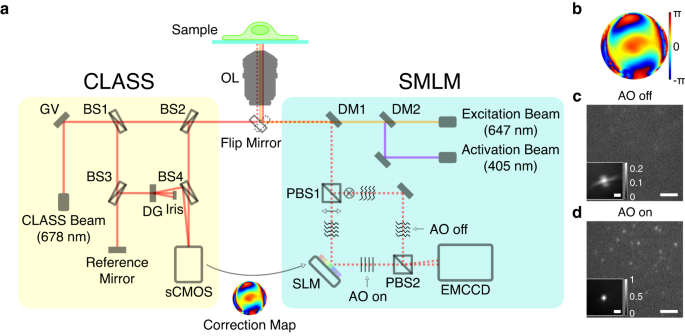This scientific illustration is an intricate technical diagram brimming with detailed nomenclature and measurement scales. At the top left, the diagram is divided into two primary sections labeled "class" and "SMLM." The "class" section features a tan box containing various labeled components such as GV, BS1, BS2, BS3, BS4, DG, iris, and a reference mirror, alongside a beam designation of 678 nanometers (nm). A yellow square marked as cCMOS and a gray item denoted as OL with a flip mirror function are also present.

On the right, the blue "SMLM" section includes beams like the excitation beam at 647 nm and activation beam at 405 nm for luminous and radiation wavelength measurements. Displayed is a glowing, multi-colored globe (item B) with colors ranging from blue to red to indicate a potential heat index, scaled from -TT to TT, with zero in the middle. Other notable elements in this section include smaller graphical representations such as a correction map, a gray square (item C) with a representative image, and a gray box (item D) labeled with scales of zero to 0.2 and zero to 0.501, respectively.

Additionally, this section features numerous labeled items like DM1, DM2, PBS1, PBS2, SLM, AO, EMCCD, and AOOFF, possibly signifying various parts of the mechanism or system at play. Connecting these sections is a centrally placed flip mirror, highlighted with the gray item OL, bridging the intricate components on either side. The diagram also utilizes a vibrant palette including yellows, blues, reds, greens, oranges, purples, grays, whites, and blacks to variously denote different elements and their relationships within the system.